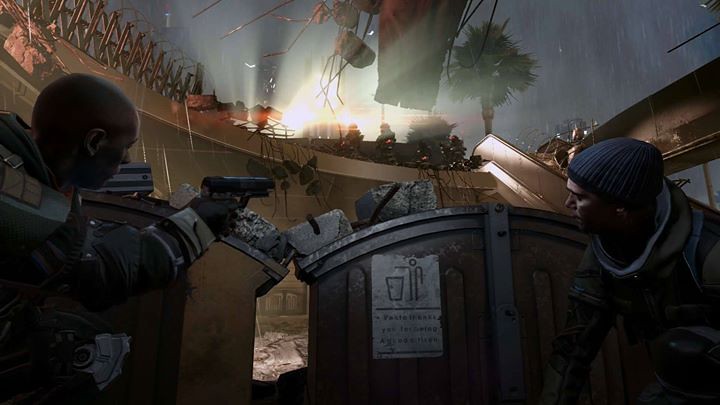This is a screenshot from a video game, showcasing a chaotic, war-torn environment that resembles the interior of a bombed-out church. The image is rectangular, illustrating two human figures positioned in the foreground amidst broken structures and debris.

The figure on the left is mostly seen in silhouette, identifiable by his bald head and the pistol he's aiming off to the right. He appears crouched behind some rubble or building pieces for cover. On the right side, another figure is crouched down behind a wooden object, partially obscured by the surroundings. Both figures seem to be clad in uniforms, indicating a military or combat setting.

The background reveals a partially destroyed roof with hanging rebar and concrete debris, suggesting a recent explosion or heavy damage. A palm tree is incongruously situated indoors, hinting at the severity of the destruction. Additionally, there is a bright light in the distance, and elements like barbed wire, a staircase, and various metallic fragments are scattered throughout the scene, amplifying the chaotic atmosphere.

Between the two figures, there's a small sign that pertains to waste disposal, which seems out of place amidst the conflict. Further in the background, on top of a wall, additional figures can be seen, apparently armed with rifles and searching for targets, adding to the tension and sense of danger in the setting.